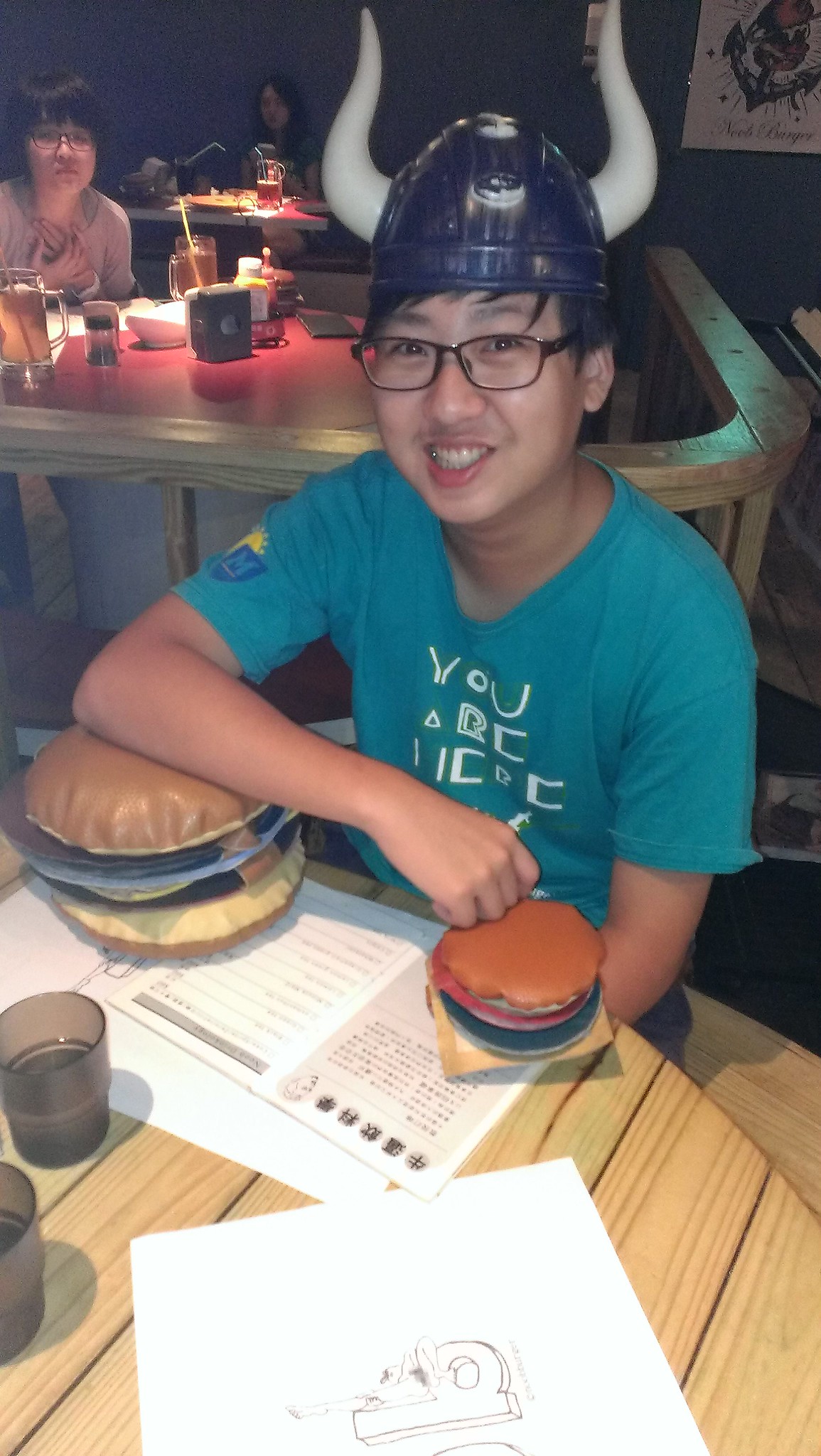In this vibrant photograph taken in a restaurant, an Asian teenager sits at a wooden table adorned with a playful Viking hat, blue with white horns protruding. He wears glasses and a turquoise t-shirt that displays the phrase "You Are Here" in white text. His broad smile adds a cheerful atmosphere to the image. In front of him lies a menu, and to his side is a large plush hamburger pillow, which his elbow rests upon. His hand lies over a smaller imitation burger, indicating that these are not actual hamburgers but decorative elements. The backdrop reveals a lively setting with other Asian patrons, including a woman with a drink and another person at a distant table. The overall scene is vibrant and filled with whimsical details, highlighted by the boy's joyous expression and quirky headgear.